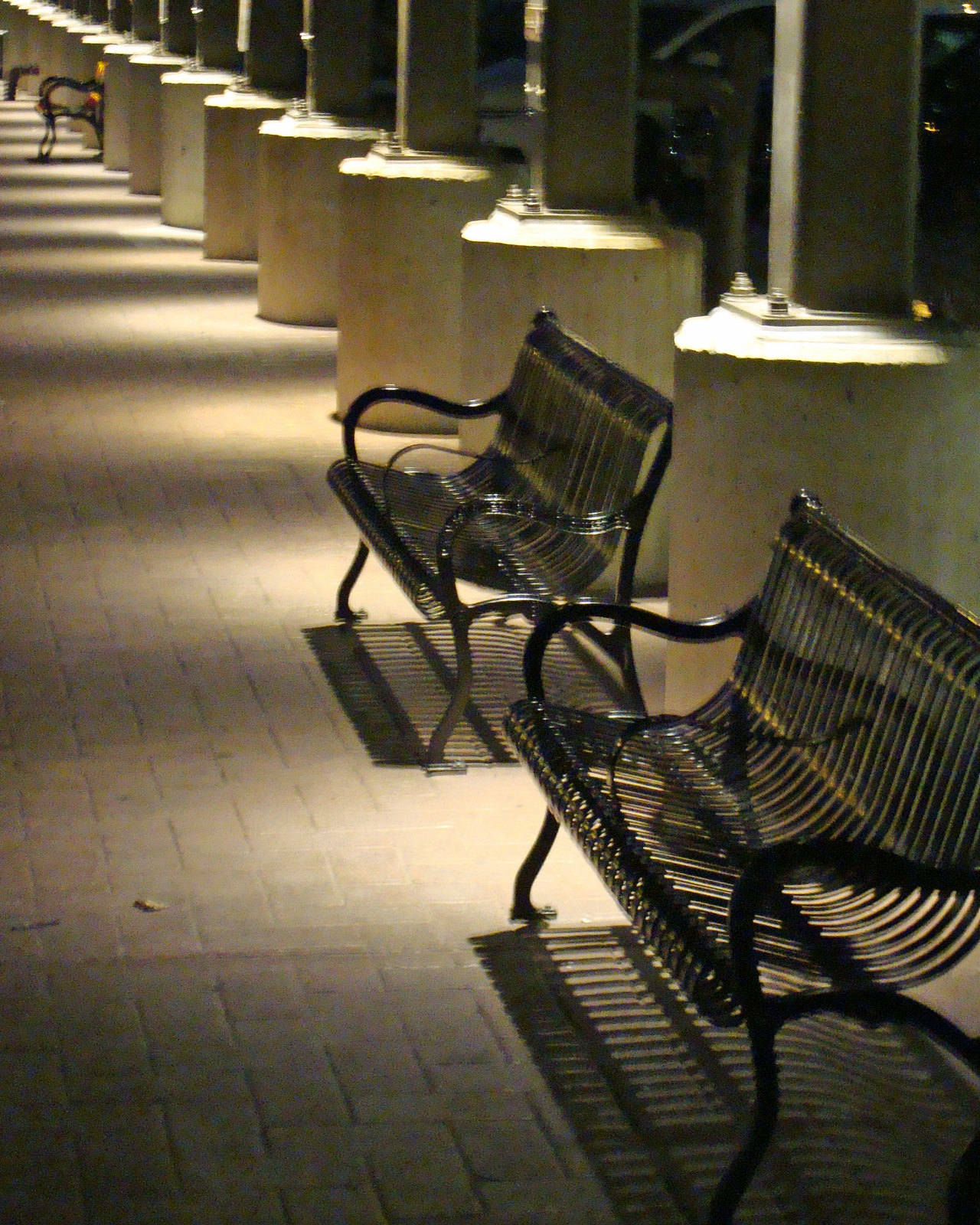The night-time photograph captures a detailed outdoor scene on a brick-paved pathway, prominently featuring two black wrought iron benches with intricate curves and slats creating patterned shadows on the ground below. Each bench is equipped with three armrests—two at the ends and one in the middle—designed to prevent people from lying down. Behind the benches, large circular concrete pylons with metal supports extend upwards, suggesting an unseen overhead structure. Dim lights above the benches cast faint, elongated shadows, enhancing the nighttime ambiance. In the distance, the brick pathway continues where two more benches are faintly visible, adding depth to the image. Farther back, the presence of a person or object walking hints at the life beyond this quiet, structured urban space.